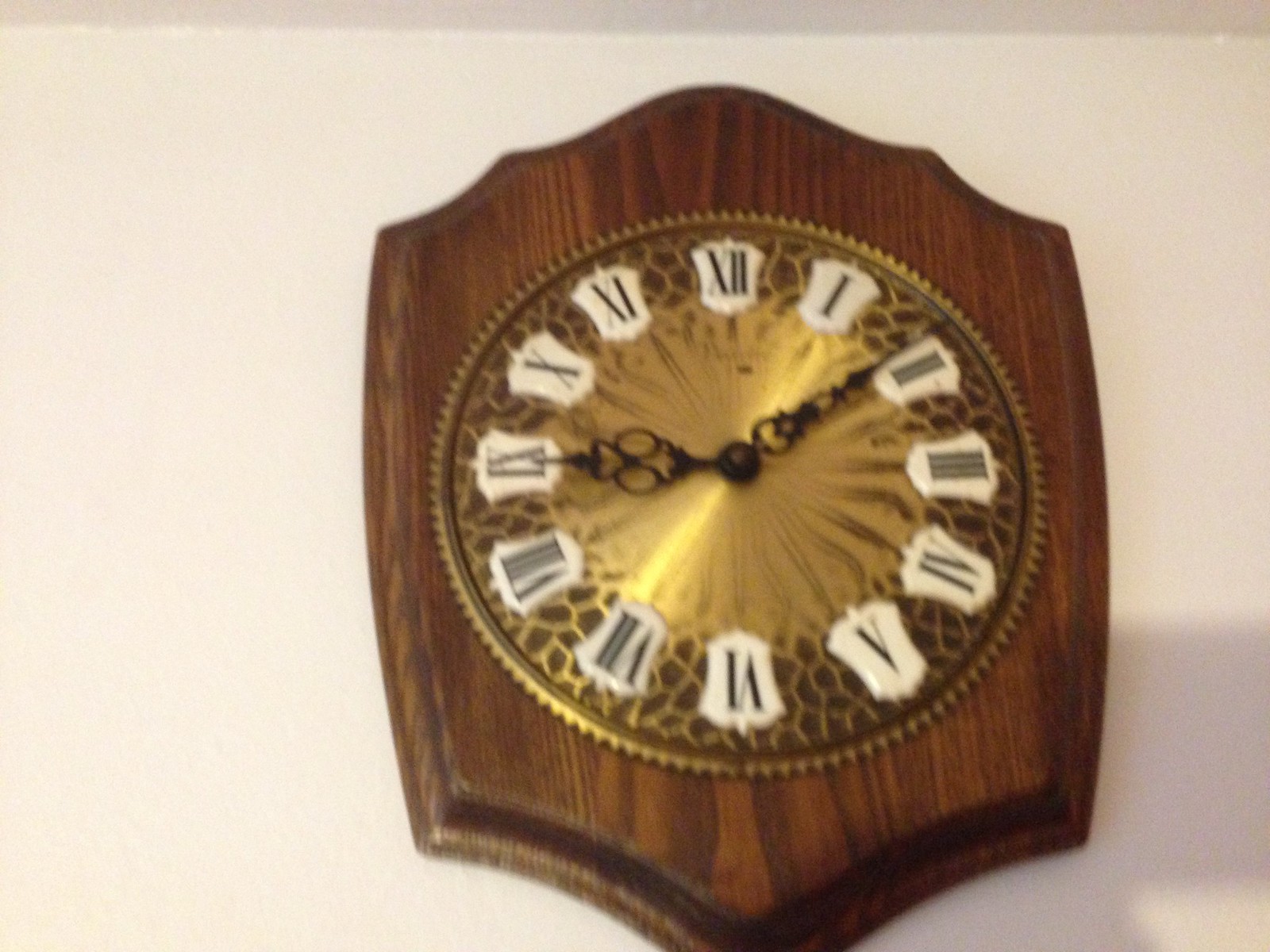The image depicts a detailed and ornate wall clock mounted against a plain white or light gray wall. The clock is enframed by an intricately carved wooden mount, stained in a rich brown hue. The overall shape of the wooden case is reminiscent of a badge, with a distinctive V-shape at the bottom and a ruffled, decorative edge at the top. The clock face itself is a striking golden color, embellished with what seem like radiating lines or intricate patterns, giving it an almost saw blade-like appearance around the edge. In contrast to this gold face, the numbers marking the hours are Roman numerals, elegantly displayed in black and set against raised white spots for a clear and classic presentation. The hour and minute hands of the clock are also black, featuring elaborate designs with loops and pointed tips that enhance the timepiece's intricate aesthetic. This elegant clock, with its harmonious blend of gold, black, and wood tones, adds a touch of classic refinement to any room.